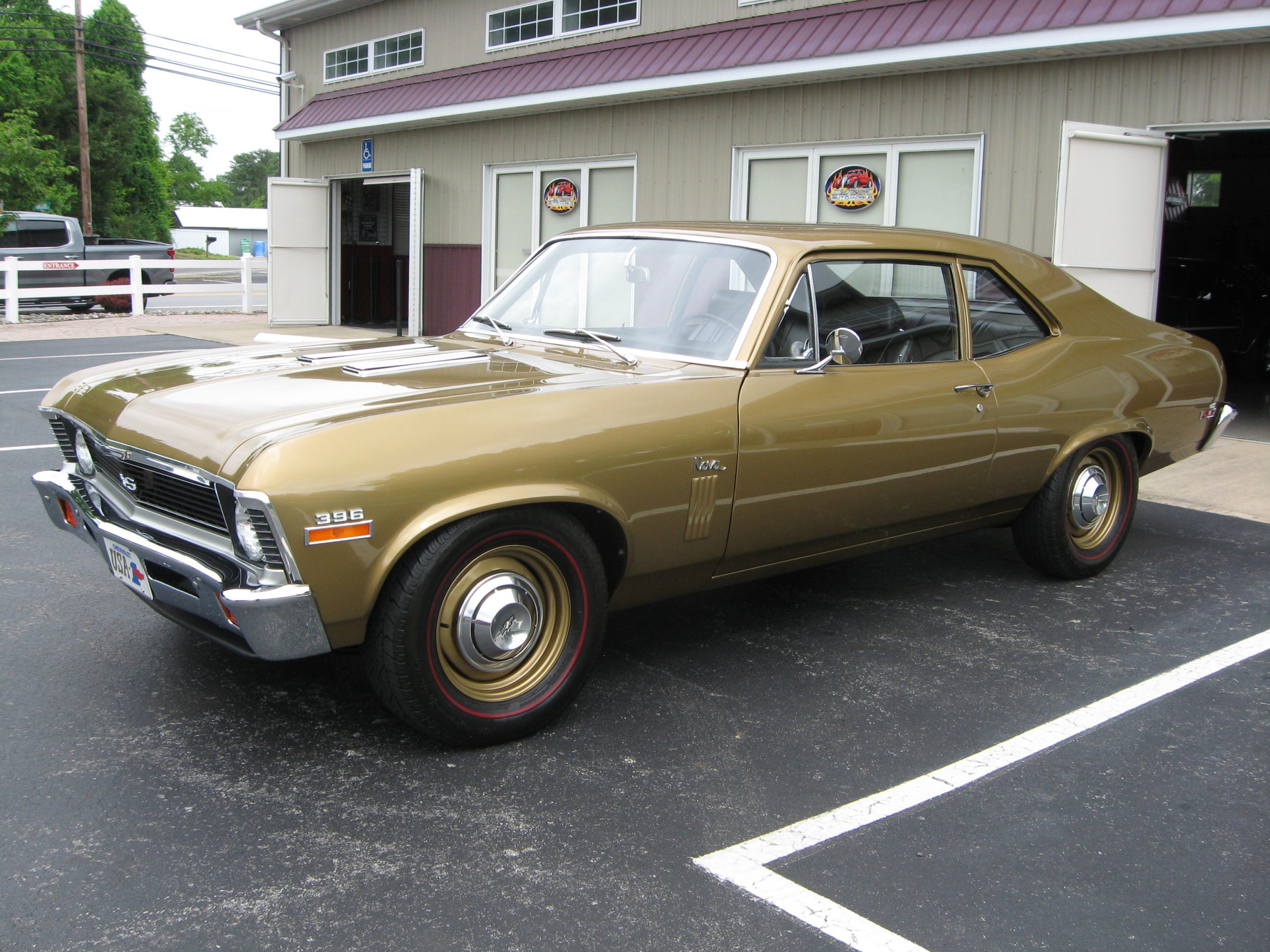This photograph captures a classic 1970s muscle car, possibly an SS Camaro, parked in an outdoor parking lot of what appears to be an auto repair or collision shop. The vehicle is a striking gold or bronze color with matching gold chrome rims and a distinctive red outline running along the circumference of the tires. The number "396" is prominently displayed on the car's side, indicating its engine size. The front grille features an 'S' emblem, and the car has a chrome grill, bumper, side mirrors, and hubcaps. The setting is an overcast day, with the car slightly angled to the left and the photo taken from adult human height. The building behind it is a beige prefab structure with two manually operated garage doors, one on each side, and a red metal roof. There is a white fence and a road in the distance, beyond which another building and some trees are visible. A more modern gray truck is parked behind the fence, further emphasizing the scene's rural, industrial feel.